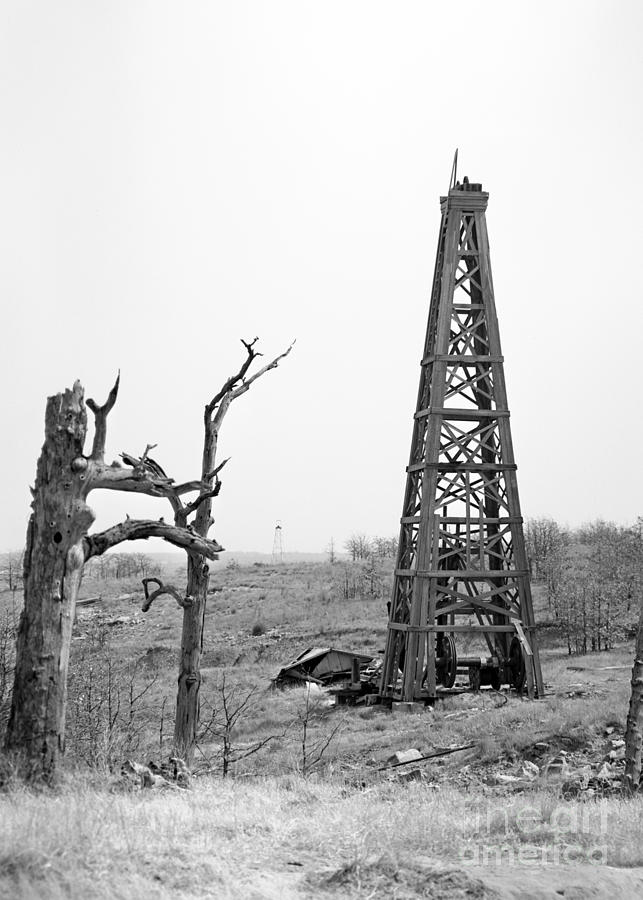The black-and-white photograph, labeled "the art America," captures a desolate scene dominated by an abandoned, A-frame steel tower, possibly once a watchtower or drilling structure. The tower, with its triangular shape, starts wide at the base and narrows as it rises, featuring wood and steel latticework between each level. Surrounding the tower is a fenced-in grassy field, where the grass appears dried out and lifeless. The area is littered with debris, suggesting a past fire or long-term neglect. To the right, two trees stand out: one partially destroyed as if struck by lightning, and the other completely barren. Additional sparse trees and broken tree trunks are visible in the background, adding to the bleak atmosphere. Far in the distance, another tower similar to the primary one can be seen, reinforcing the theme of abandonment and desolation. The overall mood of the photograph is stark and empty, evoking a sense of long-forgotten utility and life.